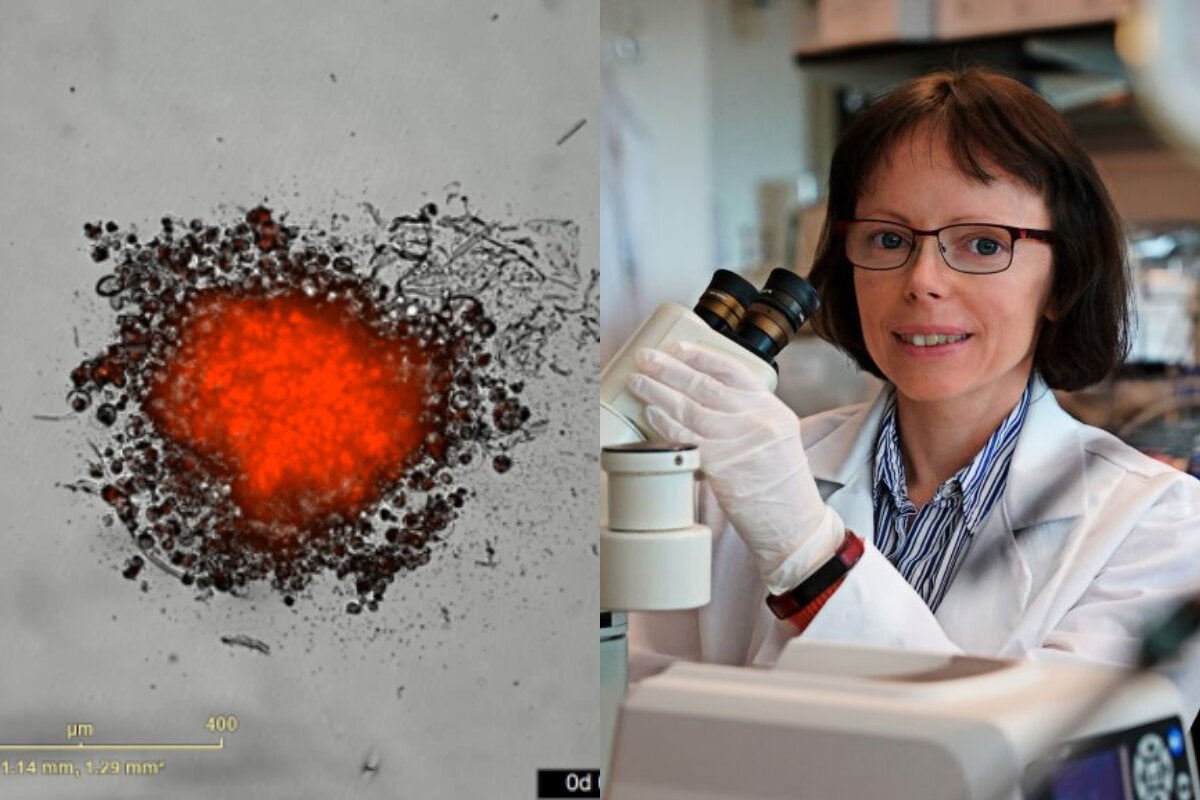The image features a dual photorealistic snapshot. On the left side, a highly magnified view captures a bright orangey-red microorganism or cell with a distinct center spot. The image also reveals a scattered pattern that may represent mold, surrounded by smaller dotted structures. A yellow scale bar at the bottom-left indicates measurements such as 114mm and 1.29mm, helping to convey the magnification level.

On the right side, a white female scientist is depicted in a laboratory setting. She is wearing a white lab coat over a blue striped collared shirt and dark gloves. She has dark brown hair styled in a bob cut, and she is smiling, appearing pleased with her analysis. The scientist is holding a microscope, suggesting she has just finished examining the microorganism displayed on the left. The background includes additional laboratory equipment, reinforcing the scientific context of the image.